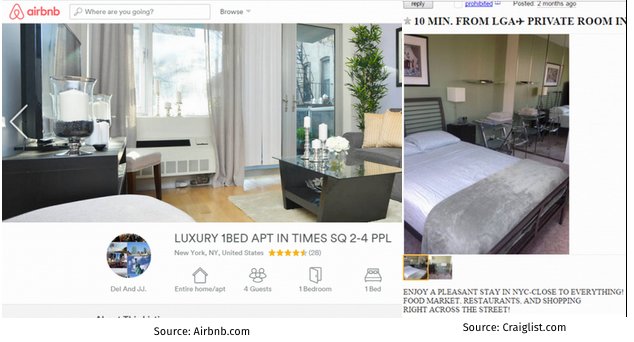This is a screenshot of the Airbnb website, identifiable by the distinctive Airbnb logo at the top left corner. The logo, colored in red, features a triangular shape with a light bulb-like figure inside. Directly to the right, there is a search bar prompting users with the question "Where are you going?" and a browse drop-down menu for navigating the website.

Below the header, the main content showcases an image of a room listed on Airbnb. The room appears to be modern and well-appointed, featuring an air conditioning unit, a door with a glass see-through window, gray curtains, and a large flat-screen TV. A notable decorative element in the room is an oversized candle holder positioned near the TV.

Accompanying the image is a detailed description of the listing: "Luxury One Bed Apartment in Times Square." The apartment is suitable for 2 to 4 guests and is located in New York, New York, United States. It has received a rating of 4.5 out of 5 stars, based on 26 reviews. The listing is hosted by users Dell and JJ.

Additional icons and text at the bottom provide further details about the property: it is an entire home/apartment, accommodates up to four guests with one bedroom and one bed. On the right side of the description, there is a note indicating that the apartment is ten minutes from LaGuardia Airport (LGA) and offers a private room, which indicates this particular feature might also be listed on Craigslist.